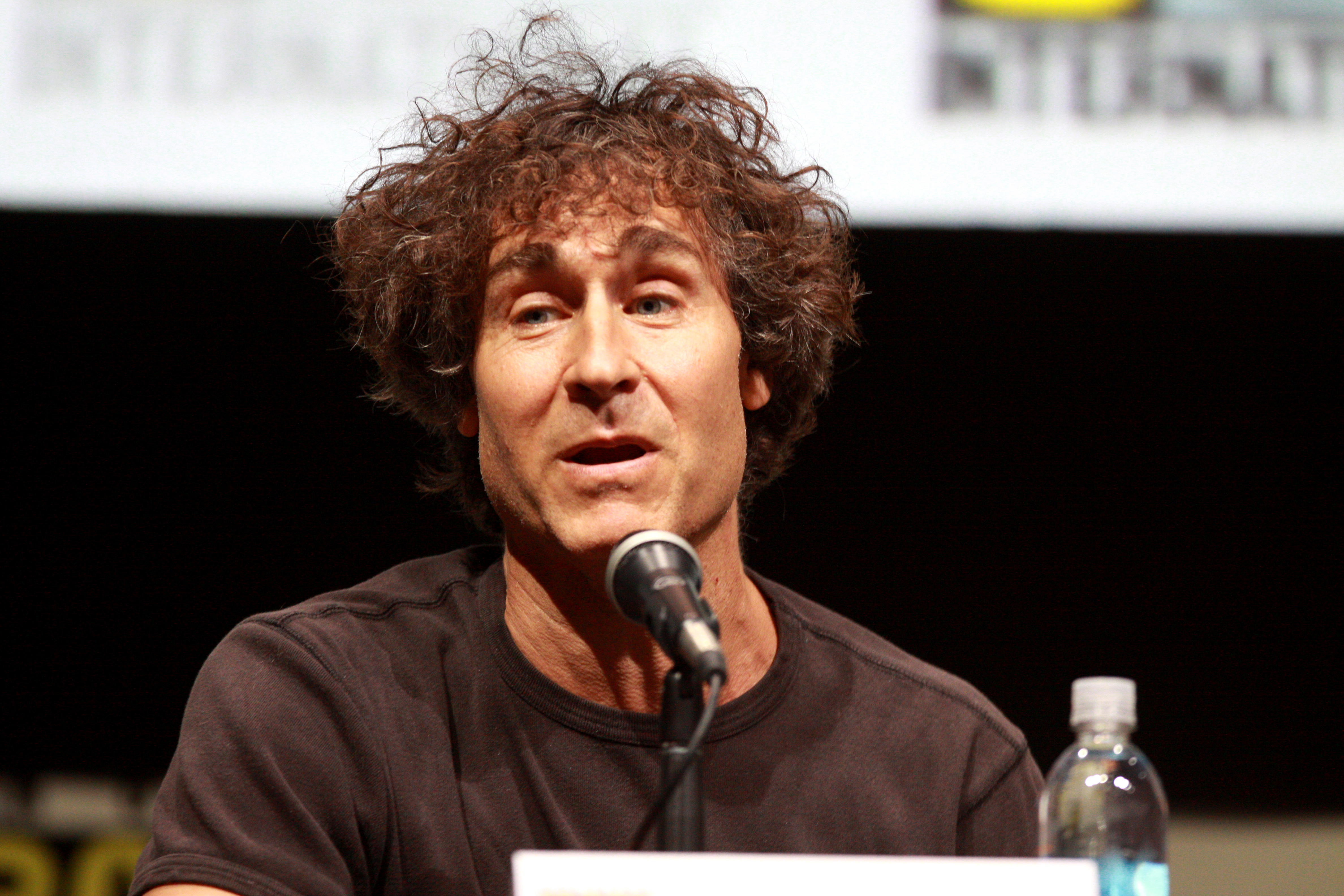The image features renowned author Neil Gaiman sitting at a table, speaking into a wired microphone placed in front of him. He is dressed in a short-sleeve, brown cotton t-shirt. Gaiman, identifiable by his distinctive squarish face, unruly short brown hair, and green eyes, has his mouth slightly agape as if he's addressing an audience or answering a question. To his left sits a single-use plastic water bottle. In the background, there is a blurred billboard-like backdrop, with the bottom half in black and the top half in white, which contains some illegible black lettering. The focus remains sharply on Gaiman, emphasizing his central position in the image.